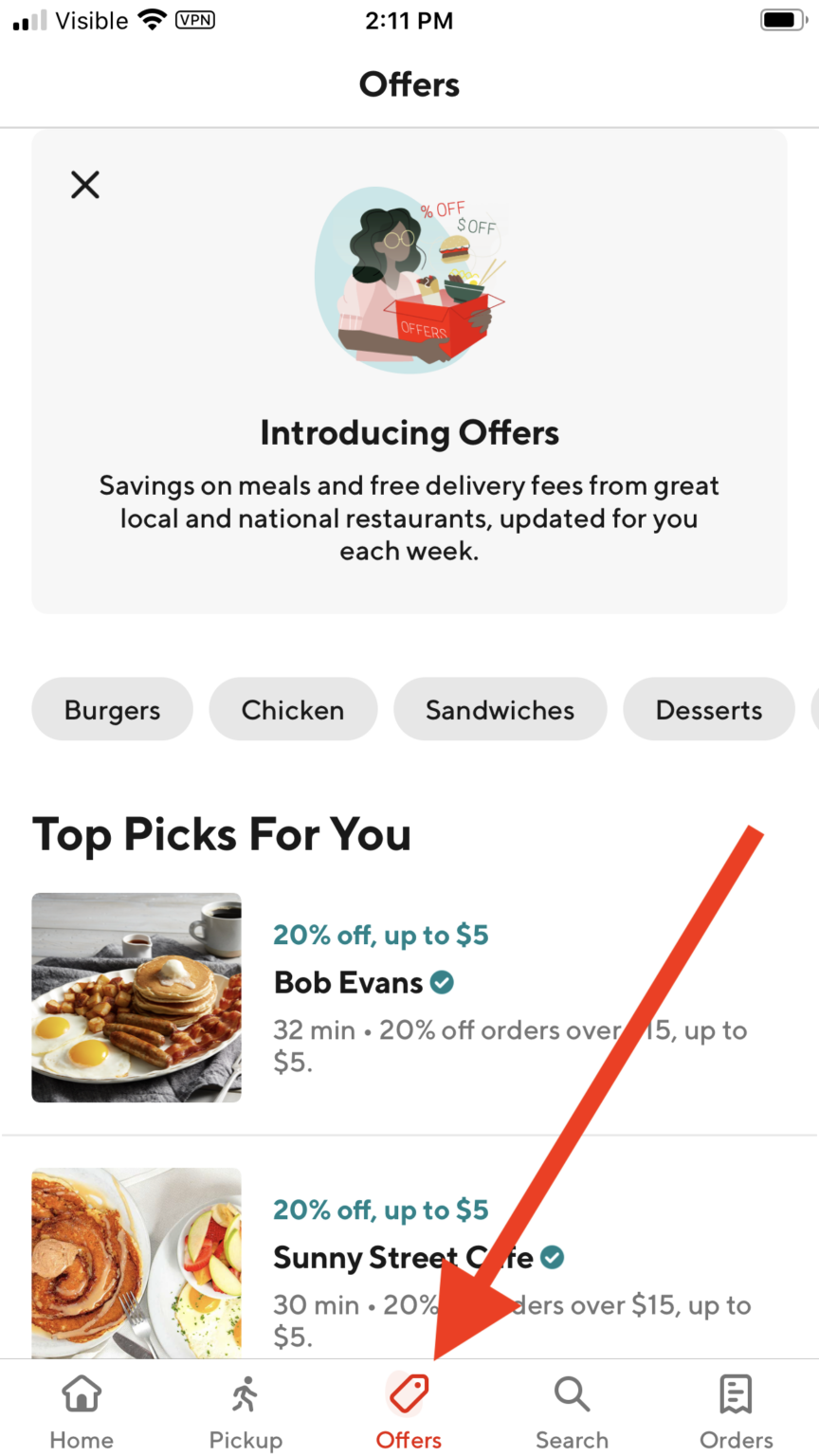This is a screenshot of a smartphone displaying the DoorDash app on the "Offers" page. At the very top of the screen, the phone's status bar is visible, displaying battery life, data signal strength, VPN icon, and the current time, which is 2:11 PM.

The DoorDash app interface starts with the menu bar at the bottom, which includes five icons: Home, Pickup, Offers, Search, and Orders, each with respective logos. The "Offers" page is currently active, as denoted by its red color, while the other options are grayed out. Additionally, a prominent red arrow highlights the "Offers" icon, emphasizing the current page.

The main section of the "Offers" page features a graphic of a woman carrying food, surrounded by discount symbols. Below this graphic, text reads: "Introducing Offers - saving on meals and free delivery fees from great local and national restaurants, updated for you every week." 

This introduction is followed by two highlighted deals labeled as "Top Picks" for the user. The first offer is from Bob Evans, showcasing an image of a breakfast platter next to the title, with an offer of "20% off up to $5" displayed in blue font. The second deal is from Sunny Street Cafe, accompanied by a photo of cinnamon rolls and apples, offering the same discount: "20% off up to $5."